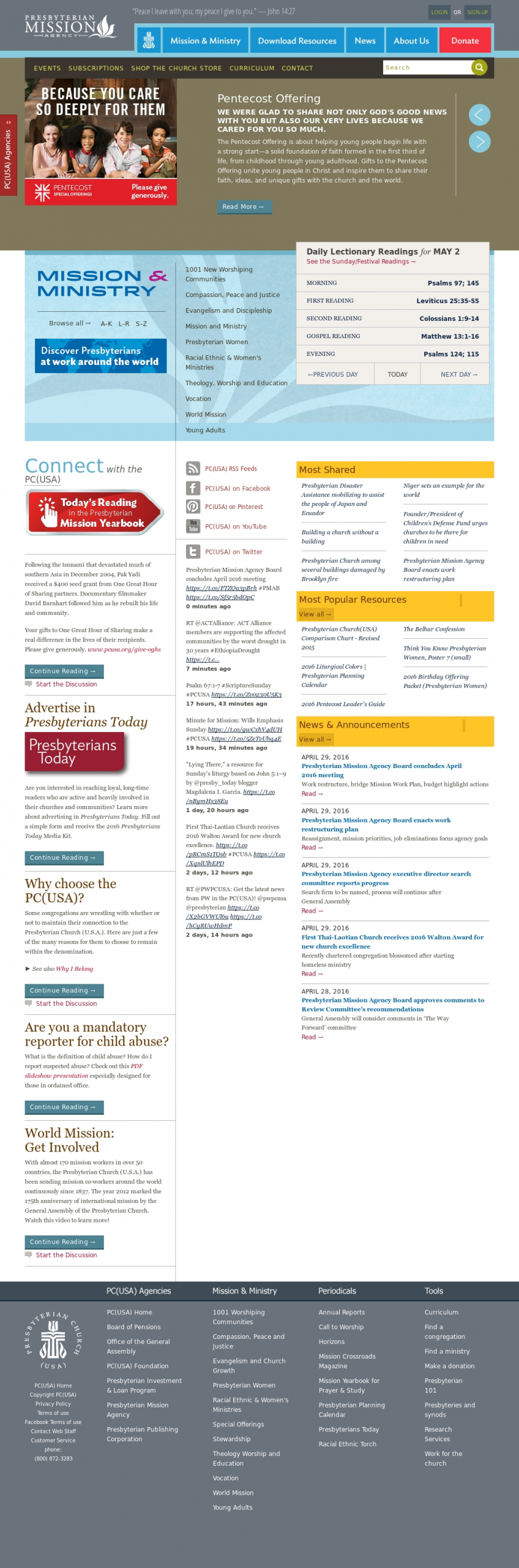In the image, we see a detailed layout of a website page against a predominantly white background, with the upper left corner highlighted against a gray backdrop featuring the "Presbyterian Mission" header. There is a prominent logo resembling a white lotus flower. To the right of this header, blue text sections labeled "Mission and Ministry," "Download Resources," "News About Us," and a red "Donate" button are neatly arranged.

Below this header, a section titled "Pentecost Offering" is prominent. It features a meaningful quote: "We were glad to share not only God's good news with you, but also our very lives, because we cared for you so much." This section emphasizes the significance of the Pentecost Offering in helping young people begin life with a strong start and a solid foundation of faith, guiding them from childhood through young adulthood.

On the left side of the page, another section titled "Mission and Ministry" invites users to "Browse All" and "Discover Presbyterians at work around the world." Below this, a feature to "Connect with the PCUSA" is visible. 

The bottom section highlights "Today's Reading in the Presbyterian Mission Yearbook" with a red button featuring a white hand icon, encouraging further exploration and engagement.